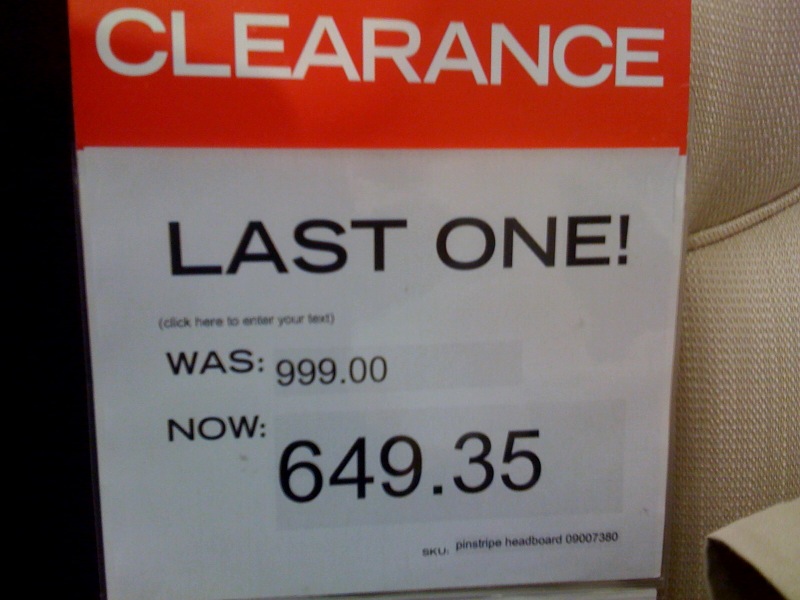The image captures a color photograph of a piece of furniture, likely a headboard, upholstered in ivory-colored, off-white fabric. The upholstery features distinct piping running horizontally across the middle, adding a touch of detail to the otherwise smooth, rounded top and straight bottom edges, typical of the armrest or top section of the furniture. The background on the left side is purely black, creating a stark contrast that directs the viewer's focus to the central elements of the image.

Prominently placed in the middle is a sale tag or label. The top portion of the tag is red and boldly reads "CLEARANCE" in all capital, white letters. The lower section of the tag is white, featuring black lettering with several pieces of information. It excitedly announces "LAST ONE!" followed by a peculiar placeholder text, "Click here to enter your text." Below that, the price is indicated, showing that the item was originally priced at $9.99 and has been significantly reduced to $6.49.35. In the bottom right corner of the tag is a SKU number for inventory purposes. Additionally, the tag identifies the item as a "Pinstripe Headboard," along with a small item number.

The overall meticulous detail in both the description of the piece and the clarity of the sale information serves to effectively communicate the nature and current sale status of this furniture item.